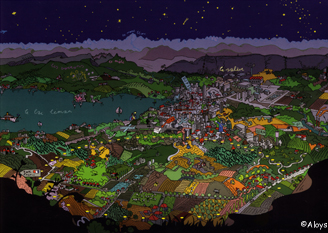This rectangular animated image depicts a vibrant, colorful topography viewed from above. The scene features a contrasting palette with diverse elements. The sky at the top of the image is dark purple, dotted with yellow stars and includes a small streak representing a shooting star. Beneath the sky, the topography shows various layers of hills and mountains in shades of purple, maroon, and gray, transitioning into green hills. These hills slope downward into an area representing a settlement or urban locale, possibly illuminated with numerous lights arranged in an oval shape. Water bodies appear both centrally and at the bottom of the image, with the lower corners enveloped in darkness, suggesting deeper waterways. The bottom edge of the illustration has a line of land extending from left to right, curving from the left side to the middle before ascending again. Within this scene, the urban area at the middle highlights buildings and structured spaces with varying colors, giving the setting a lively look, reminiscent of a bustling cityscape noted for its dynamic vibe akin to that of "The Simpsons" animation style. Lastly, in the bottom right, white letters form an inscription, albeit slightly unclear, that reads 'CALOYS.'